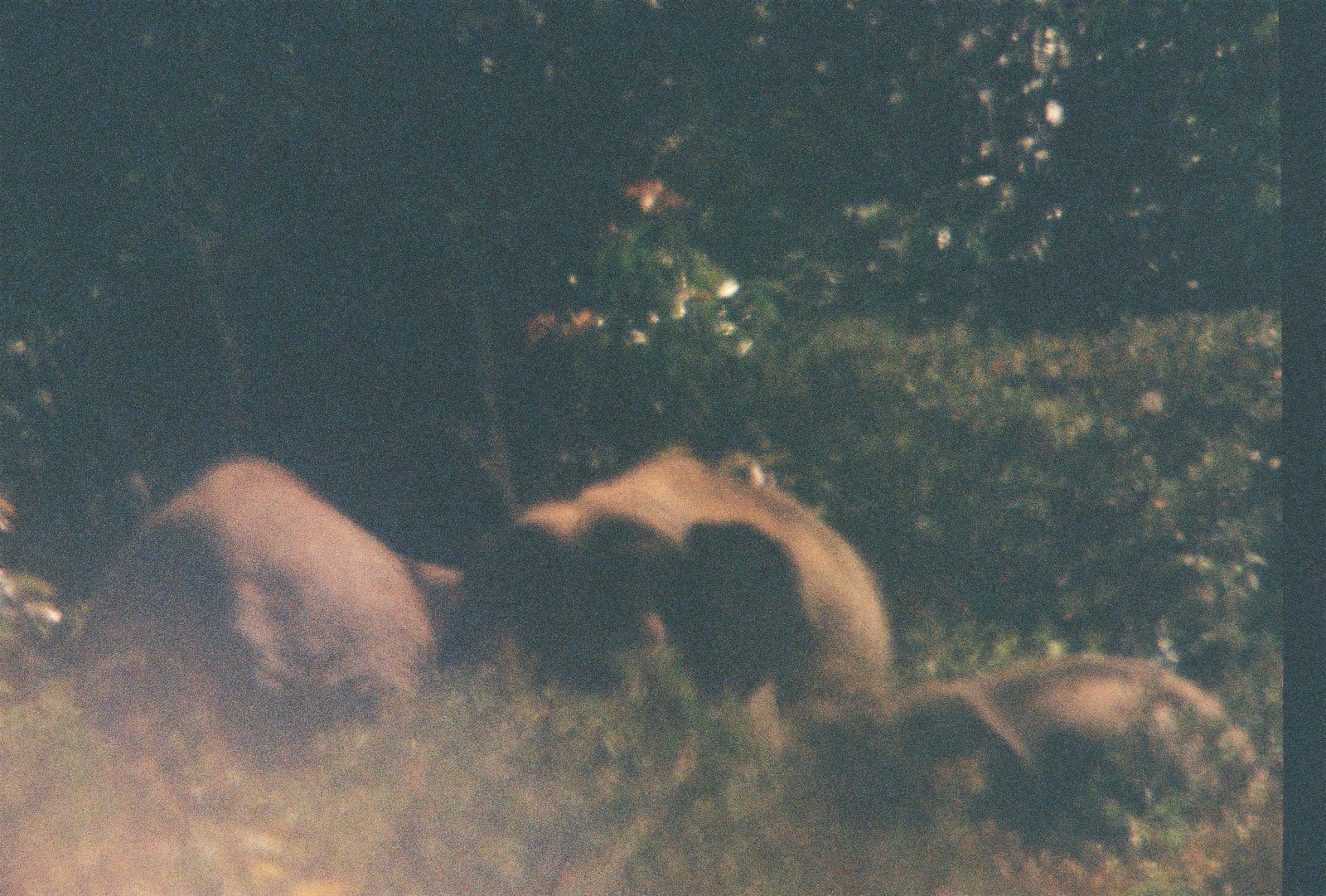In this obscure and blurry photo, set against a dark green forest backdrop, there appear to be three elephants nestled in the green and yellowish bush. The image is grainy, suggesting it might be an undeveloped film photo, adding a mysterious yellow tint at the bottom. The two larger elephants are positioned on the left, with one of their grey, humped backs and possibly an ear and a tail slightly visible, despite the photo's out-of-focus nature. The smaller elephant on the right, likely a baby, shows a side view of its head and the ridge of its spine, protruding upwards. The scene is enveloped in tall brush and branches, enhancing the sense of secrecy and the natural habitat of what looks like a family of elephants.